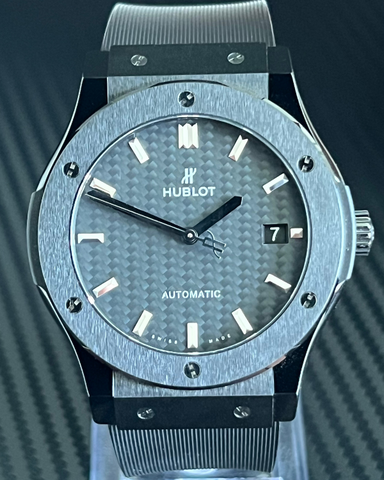This image showcases a luxurious Hublot watch on a stylish blue and gray diagonal-striped background. The watch itself features a high-quality gray wristband and a blue and gray dial, which contains minimalist hour markers instead of traditional numbers, with a thicker marker at the 12 o'clock position. The watch face displays a small window at the position where the number 7 would be, likely indicating the date. Notably, "Hublot" and "Automatic" are inscribed above the center and near the six o'clock position, respectively. The iconic Hublot logo, an H with a zigzag line, is prominently featured, emphasizing the brand's identity. The sleek design and sophisticated color scheme make this watch appear exceptionally elegant and desirable.